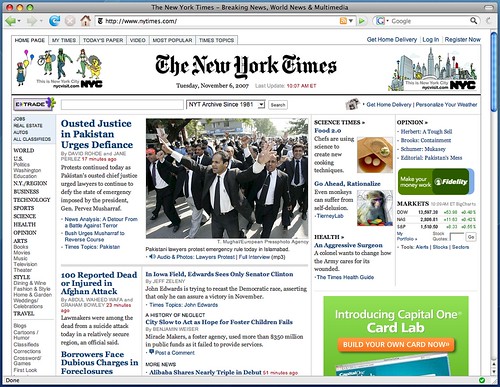The image depicts the homepage of The New York Times website, featuring a gray-bordered header at the top with the text "The New York Times, Breaking News, World News, and Multimedia." Below the header, a navigation bar includes a green left-pointing arrow, a blue refresh button, a home icon, and an address bar displaying "www.nytimes.com." To the right of the address bar, a Google search bar is visible.  

Following this, there is a menu with options labeled "homepage, My Times, today's paper, video, most popular, Times topics." On the far right side of the menu are links for "get home delivery, log in, register now."  

Beneath the menu, The New York Times logo is prominently displayed in large, bold black letters. To the right of the logo, an illustration showcases the New York City skyline with "NYC" written underneath it. 

At the center of the image, a photograph captures a group of people marching through the streets dressed in business suits and ties. The caption above the photo reads "Outer Justice in Pakistan, Urgent Defiance." Below the image, another headline states, "100 Reported Dead or Injured in Afghan Attack."